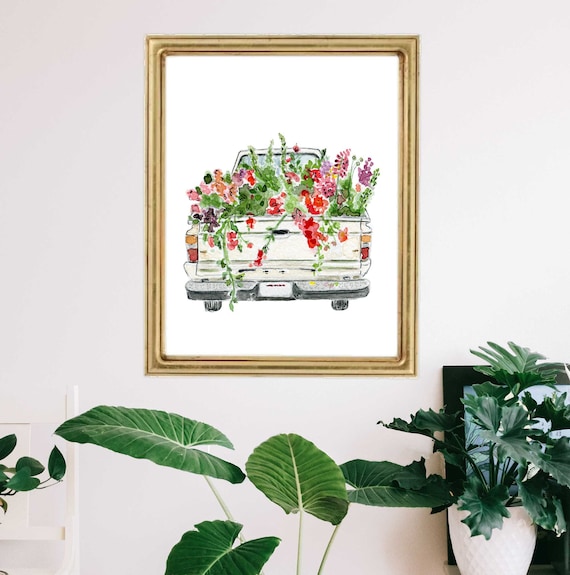The photograph captures a serene, minimalistic room with pristine white walls, focusing on a gold-framed painting that hangs centrally. The painting within the golden frame portrays the back of a white pickup truck driving away, its bed overflowing with vibrant flowers in a palette of reds, pinks, purples, and lush greenery. The truck's taillights and the densely packed flowers tower above the cab, creating a striking contrast against the white, blank background of the painting. In the foreground, the tops of several plants are visible, adding a touch of nature to the room. On the bottom left, a white chair is partially visible, while the bottom right corner features a white planter holding a plant, which slightly obscures a black wooden frame. The overall composition of the room is clean and uncluttered, contributing to the overall aesthetic appeal.